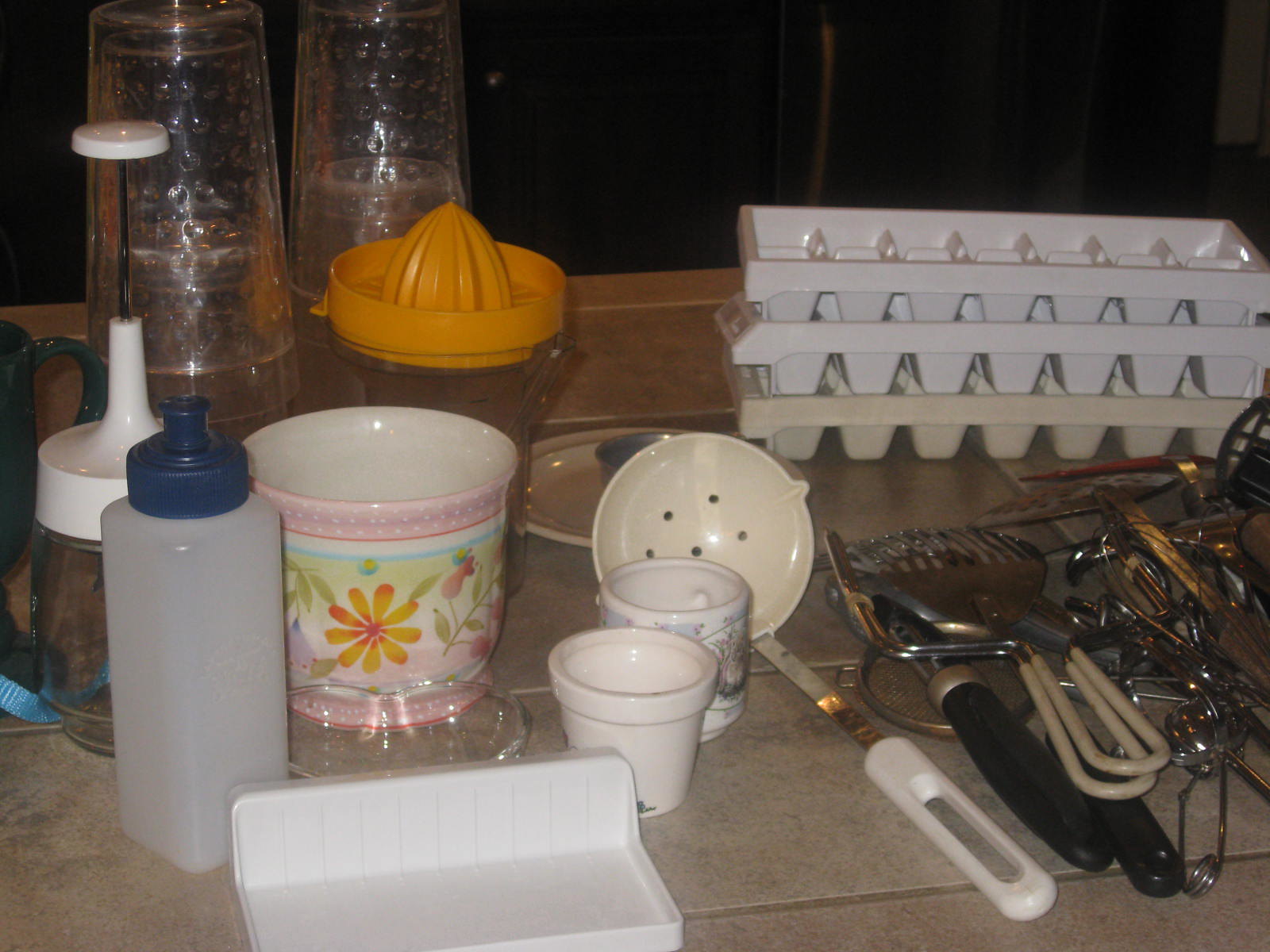In the image, a variety of kitchen utensils and items are arranged on a beige tiled countertop with light grout. Towards the back, three ice trays are neatly stacked on top of each other. On the left side, four glasses are placed upside down in two stacks next to an orange squeezer. Positioned in front of the glasses is a slap chopper, with a plastic bottle sitting directly in front of the chopper. In front of the plastic bottle lies a white butter tray, with two small ceramic cups located behind it. A ladle is situated to the right of the butter tray, surrounded by various pieces of silverware and other kitchen utensils, all clustered together. The background features a dark wooden wall, possibly part of a door equipped with a brass doorknob.